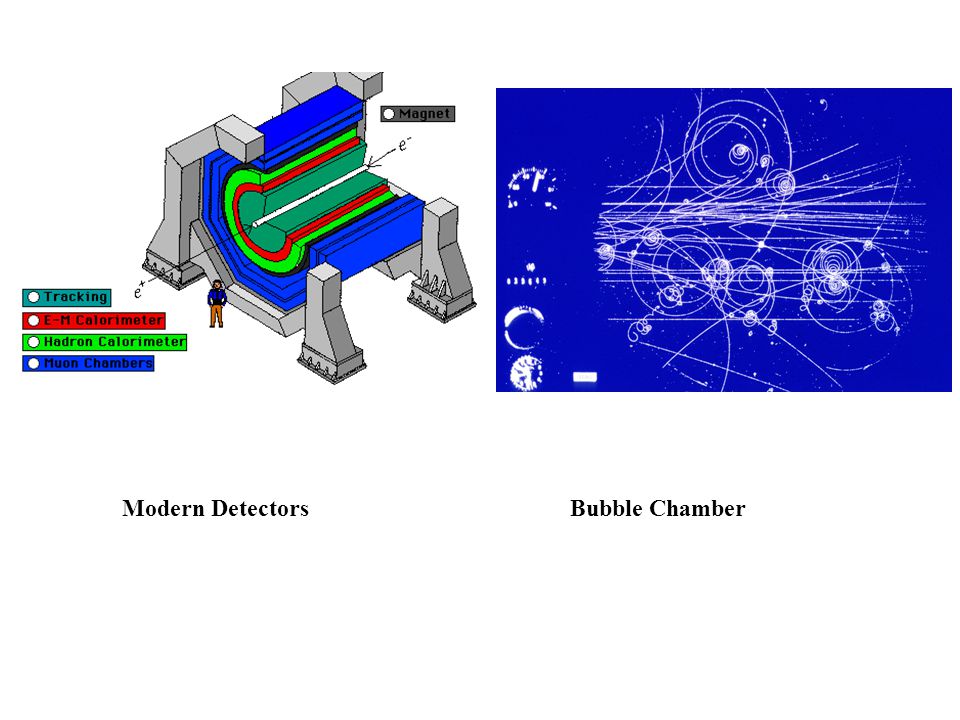The image depicts a diagram of a particle accelerator and its components, divided into two parts: a "Modern Detectors" section on the left and a "Bubble Chamber" section on the right. 

On the left, the "Modern Detectors" section features a cutaway drawing in a style reminiscent of Microsoft Paint, showing a layered structure, akin to a jawbreaker, with a small human figure included for scale. The structure is composed of concentric layers, each distinctly colored and labeled. Starting from the innermost part, there's a white pole (Magnet) marked with positive (E+) and negative (E-) ends. Surrounding the magnet is a teal blue-green area labeled "Tracking," followed by a red layer labeled "EM Calorimeter," then a lime green layer labeled "Hadron Calorimeter," and finally, a dark blue layer labeled "Muon Chambers" forming the outermost part. The entire assembly is encapsulated within a gray square structure with clamp-like features that support the inner components.

To the right, the "Bubble Chamber" section displays a blue schematic filled with intricate white lines, circles, and squiggles, resembling a constellation map or a readout from the particle accelerator. This schematic includes various circular patterns and what appears to be a speedometer with numeric measurements on the side. The contrast between the modern, detailed cutaway on the left and the complex, abstract schematic on the right emphasizes the advancement in detection technologies from the bubble chamber to modern detectors.

Together, the detailed cutaway of the modern detector and the intricate bubble chamber schematic provide a comprehensive visual comparison of particle detection techniques.